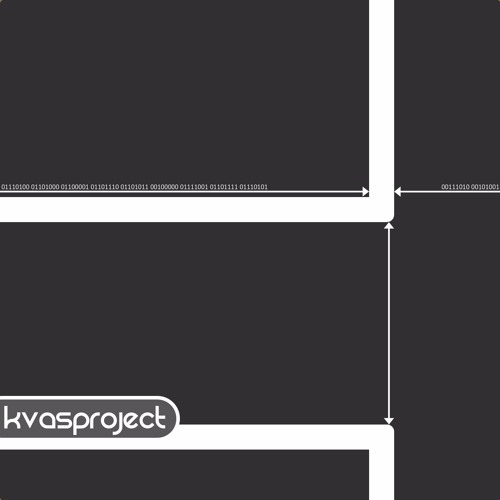A screenshot features a light gray background overlaid with several graphic elements resembling design tools possibly originating from an iPad interface. Positioned approximately 80%-75% to the right of the image, a sequence of sharply and smoothly contoured lines create a complex geometric pattern. 

From the top, a vertical line extends downward, incorporating a sharp inner corner and a curved outer corner as it makes a 90-degree turn to the left, proceeding horizontally across the screen. Below this formation, a distance marker arrow is prominently displayed. Near the bottom of the image, another line, this time inverted, runs vertically downwards after taking a right-hand turn from the left, mirroring the layout of the upper design yet inversely positioned. 

Justified in their respective positions, both the upper and lower design elements exhibit markers on their inner frames indicating precise distance measurements, further accompanied by additional markings extending beyond the frame.

In the bottom left corner, there is a gray, capsule-shaped logo with lowercase, stylized text reading "KVAS Project" written as a single word. Layered atop this intricate assembly of lines and markers is a dense matrix of binary code—sequences of 0s and 1s—spanning horizontally across the screen beyond the visible edges, adding a cryptic digital dimension to the scene.